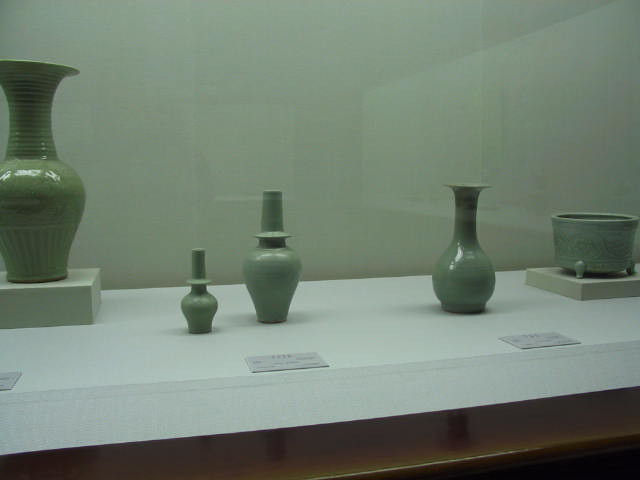This color photograph, which appears to be either taken in poor lighting or filtered for muted tones, depicts an exhibit of green pottery and vases on a creamy shelf with a wooden section at the bottom. Arranged on square pedestals, the objects include one large, glazed vase on the far left with a narrow neck and bulbous middle—partially cut off by the left edge of the image. Next to it, a smaller vase with a similar narrow neck and curvature is positioned. The middle of the display features another slightly larger vase with comparable design elements. Towards the right, a vase with a more pronounced bulbous base sits beside a deep, round green bowl on a pedestal. The background wall, possibly gray or greenish, features distinct light patterns resembling square and rectangular shapes, suggesting filtering or reflections possibly from a window. Three plaques with illegible writing lie flat in front of the pottery, contributing to the exhibit's feel. The bottom right corner of the image includes a dark section with a curious near-white line running through it. This amalgamation of details hints that the image might be AI-generated.